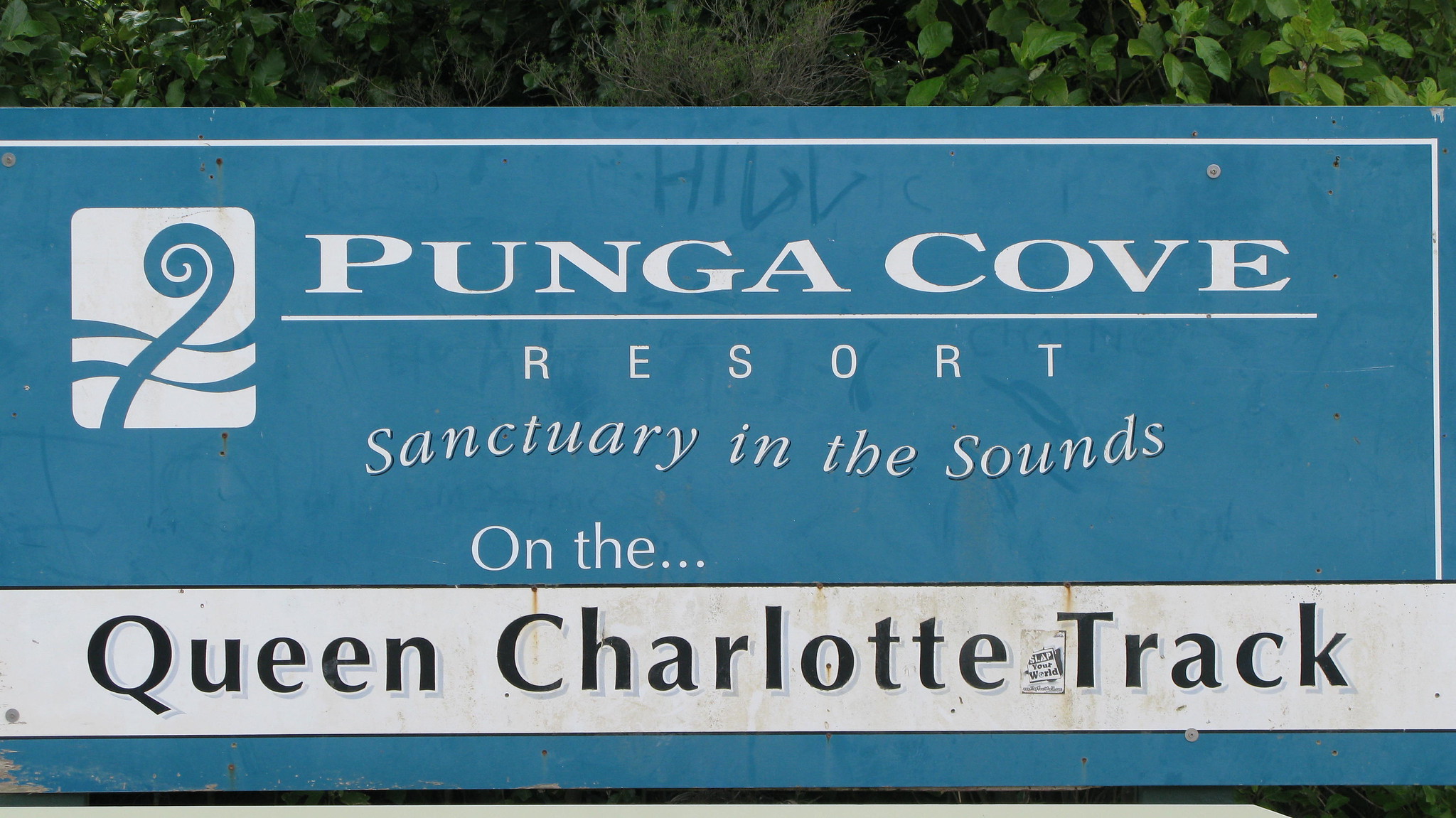The image is a rectangular photograph taken outdoors, showcasing a lush, green landscape with several trees and shrubs in the background. The focal point is a large, weathered blue sign with white and black text. The sign features a distinct logo on the upper left corner, consisting of white with blue elements designed like wave-like swirls and a curly Q. Along the top and right-hand side of the sign, there is a thin white line. In bold white caps, the main text reads "Punga Cove," followed by "Resort" with a white underline beneath "Punga Cove." Below that, it states "Sanctuary in the Sounds." Further down, a white bar with black bordering displays "Queen Charlotte Track" in black font. The blue paint on the sign appears slightly weathered, particularly along the bottom.